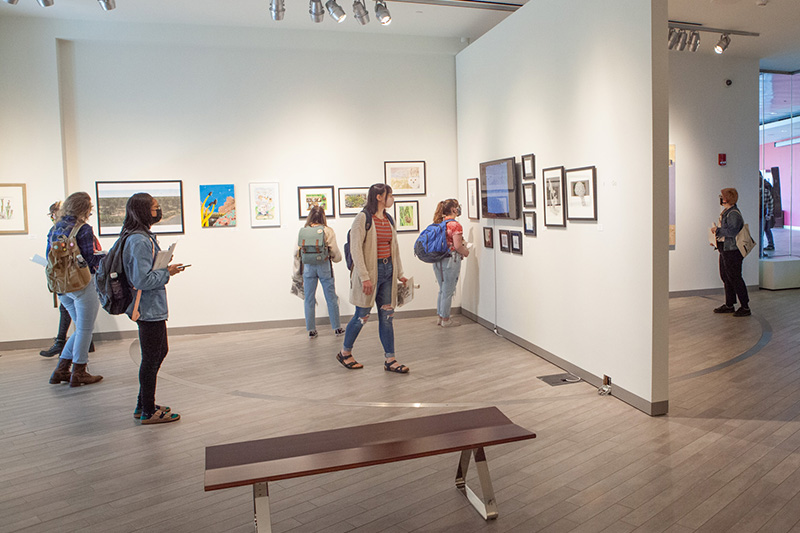The image is taken indoors, depicting a room with white walls adorned with framed art and old pictures. The lighting from above illuminates the displays, enhancing the details on the artworks. The scene appears to be in a school or an exhibit gallery. At least six people, mostly teenagers, are present, casually dressed in jeans, sandals, and some carrying backpacks. A few of them are wearing COVID-19 masks and are engaged in observing the artwork on the walls. A distinct brown bench, seemingly made of metal and featuring other materials, is positioned in the room, resting on a floor that appears to be either wood or laminate, with a gray trim at the base of the walls. In the adjacent room, additional artwork is displayed, visible through an open passage, along with a few more people examining the exhibits.